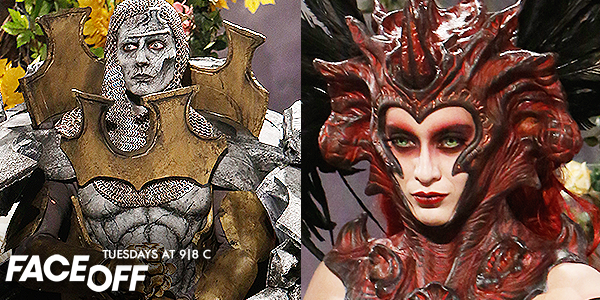The image is presented in a landscape orientation and is divided into two square segments, containing two distinct photos.

On the left, there's a character that appears to be inspired by a movie or series. This figure is a muscular man with a completely gray, almost metallic appearance. His head is covered with a silver chainmail, and he wears substantial golden armor over it. The character exudes strength and intensity. In the bottom left corner of this segment, white text reads: "Face Off Tuesdays at 9/8c".

The right-hand side features a contrasting character, a woman who resembles an enigmatic witch. She has piercing deep green eyes, accentuated by dramatic red makeup and bold red lips. Her head is adorned with an elaborate, spiky headpiece that extends over her head, chest, and shoulders. This headpiece includes horn-like protrusions, giving her a menacing and powerful appearance. Black feathers emanate from behind her, further enhancing her intimidating and otherworldly look.